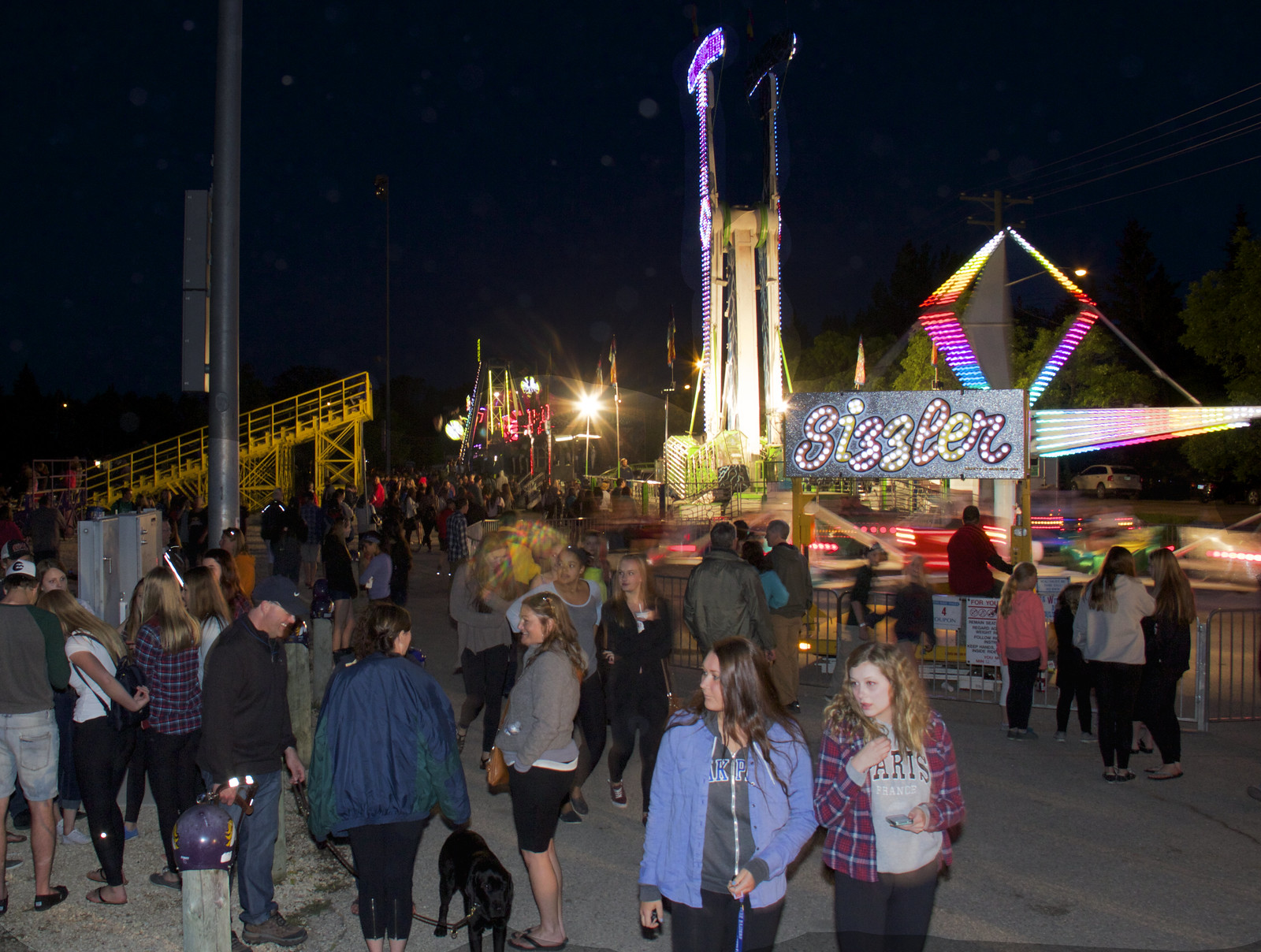The nighttime photograph captures the lively atmosphere of a bustling outdoor fair or carnival, with the dark sky serving as a backdrop to the vibrant scene. The concrete ground is filled with around fifty people, mingling, smiling, and chatting—some wearing shorts, signaling a warm night. Prominently to the right side of the image, a ride called the Sizzler stands out, adorned with a colorful cursive sign and swirling lights that depict its movement. Near the middle-left background, a yellow metallic structure, possibly a stairway or additional ride, adds to the carnival ambiance. Bright blue, pink, yellow, and red lights from various rides illuminate the scene. Among the crowd is a black Labrador, calmly on a leash beside a woman. Overall, the image encapsulates the energetic and colorful essence of a nighttime fair, bringing together diverse elements of rides, people, and vibrant lighting.